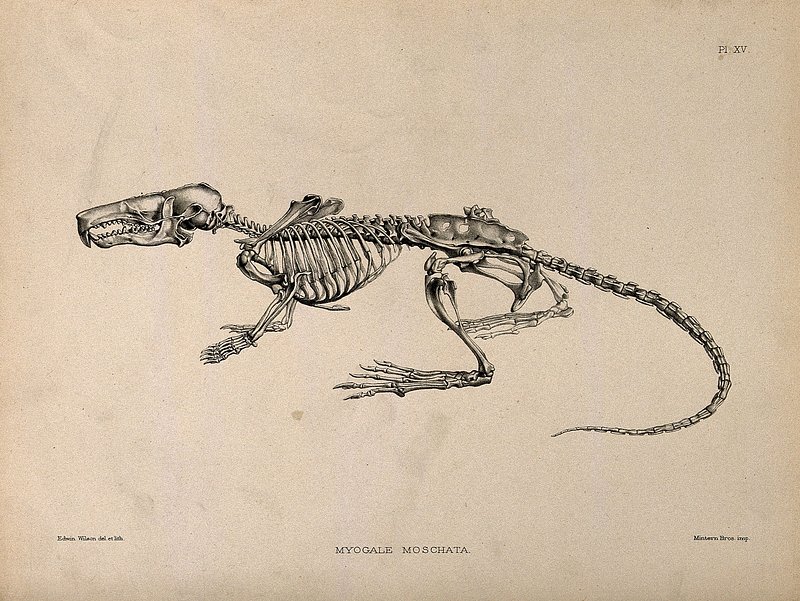The image is a detailed black and white drawing of a dinosaur skeleton positioned in a square with no border, the paper giving the appearance of old, stained parchment in a brown tone with light gray smudges and a water stain. The skeleton faces left, showcasing a long snout with visible teeth, a ribcage that narrows towards the midsection, and a long, chain-like tail that curves slightly towards the left. The animal has short legs with long, bony feet and thin toes, and equally bony hands. In the upper right corner, the text "P-I-X-V" is printed. At the bottom center, there is a caption in all capitals reading, "M-Y-O-G-A-L-E M-O-S-C-H-A-T-A," possibly identifying the species. The lower left corner features a small, hard-to-read inscription that appears to name "Edwin Wilson" or "Edwin Williams" followed by additional unclear text. The bottom right corner also contains tiny unreadable print.